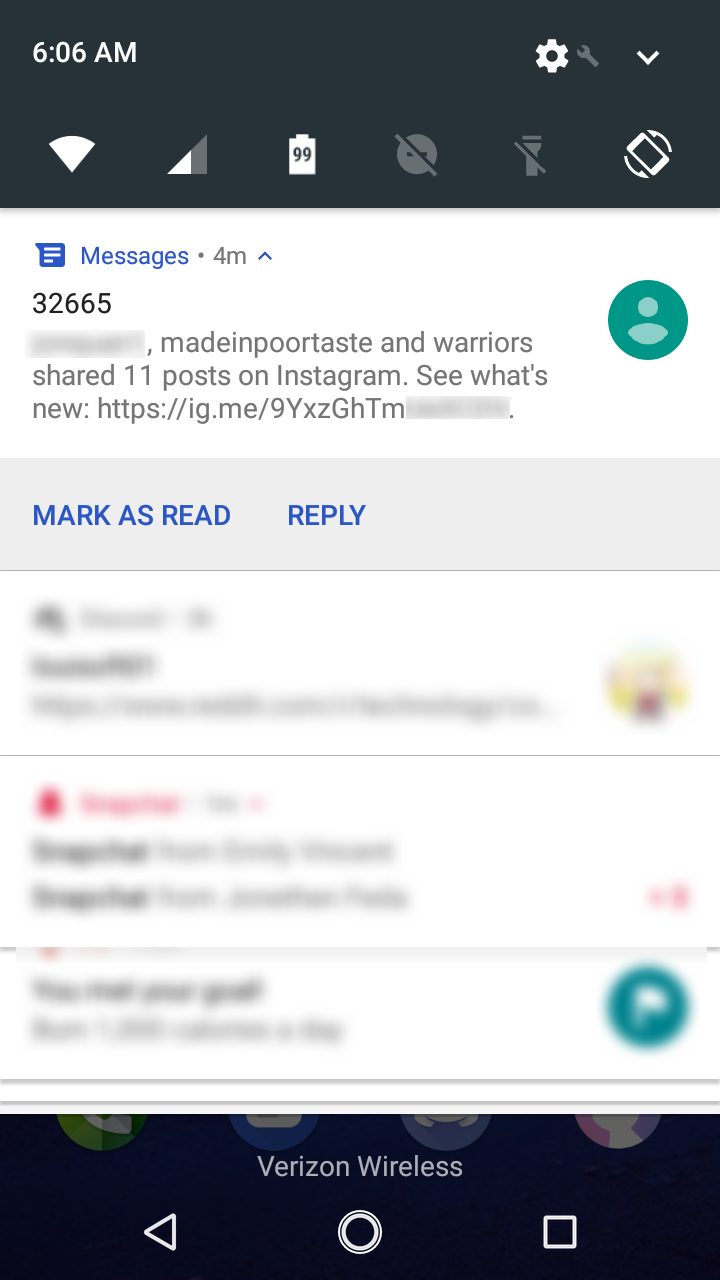The image appears to be a screenshot of a smartphone's notification center or home screen. Here's the detailed caption:

---

**Detailed Description of Smartphone Screen Image:**

The image captures a smartphone screen, possibly displaying the notification center or home screen. Here’s a detailed breakdown of its elements:

- **Top Left Corner**: The time is displayed as 6:06 a.m.
- **Top Right Icons**: 
  - A settings icon represented by a wrench.
  - A downward-facing arrow next to the settings icon.

- **Bottom Row Icons**:
  - Wi-Fi signal icon.
  - Reception bars indicating network strength.
  - Battery icon showing 99% charge.
  - An icon possibly for messages, which is crossed out.
  - A flashlight icon, also crossed out.
  - An icon for toggling the screen orientation between landscape and portrait, which is white.

- **Central Notifications**:
  - A notification highlighting "Messages" followed by "4M" (possibly indicating 4 new messages) and an upward arrow.
  - A sequence of numbers: "3, 2, 6, 6, 5."
  - A notification with the text "Made in Poor Taste and Warriors," followed by a statement "shared 11 posts on Instagram." Then, it says "See what's new:" followed by "IRL," which includes a green circle and a lighter green figure representing a person.
  
- **Actions and Other Information**:
  - A rectangle with the options "Mark as Read" and "Reply."
  
- **Additional Elements**:
  - Three more rectangles are present but appear blurred, making the content unreadable.
  
- **Bottom of the Screen**:
  - The carrier information "Verizon Wireless" is shown.
  - Three icons are visible but not detailed in description.

This descriptive caption thoroughly explains the content and layout of the smartphone screen captured in the image.

---